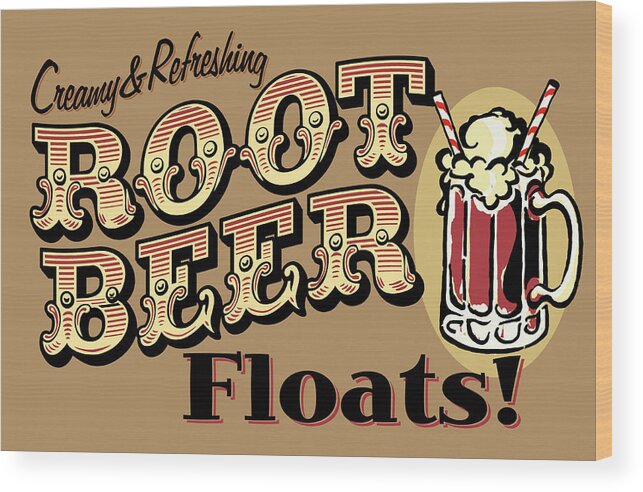The image features a rectangular wooden sign with a light brown background, providing a 3D appearance on one edge. On the right side of the sign, there is a detailed drawing of a root beer float in a brown mug, topped with a scoop of ice cream and adorned with two red and white striped straws. Bubbles are visible spilling over the sides of the mug. To the left of the drawing, the text "Creamy and refreshing root beer floats" is prominently displayed. "Creamy and refreshing" is written in an italicized cursive font, while "root beer" stands out in a bold, old-fashioned font with horizontal red and yellow stripes, outlined in black. Below this, the word "floats" is written in black with a red outline, and an exclamation point follows it, enhancing the 3D effect. The background and thickness of the wooden board are consistent with a warm brown hue, adding to the rustic charm of the sign.